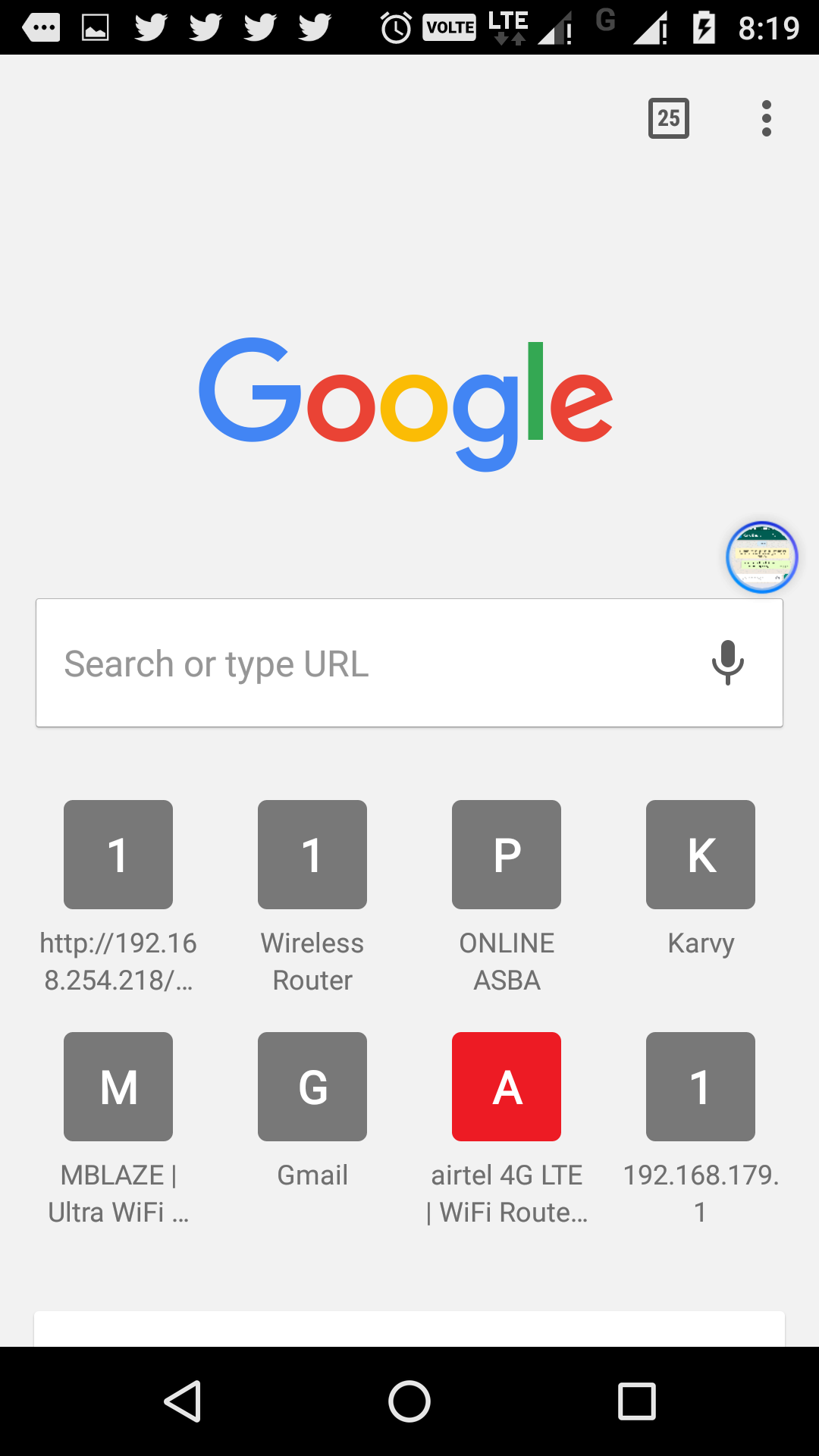In this screenshot, we see a user interface captured from a device display with a predominantly solid gray background. At the top of the screen is a black banner featuring several icons and texts. From left to right, the black banner includes four Twitter bird icons, an alarm clock, a volt icon, an LTE symbol, and the time displayed as 8:19.

Centered below the banner in large text is the word "Google." Directly beneath this word is a white search bar containing the placeholder text "search or type URL," with a microphone icon positioned to the right side of the bar. 

Beneath the search bar are four gray square icons arranged in a row. From left to right:
1. The first square displays the number "1" and underneath it reads "HTTP://192.16.8.254.218."
2. The second square shows the number "1" with the phrase "wireless router" written below.
3. The third square contains the letter "P" with "Online ASBA" or "A-S-B-A" written beneath it.
4. The fourth square bears the letter "K" followed by the word "Carvey."

Further down, the bottom row of square icons includes:
1. A gray square with the letter "M" for "Mblaze."
2. An adjacent gray square with the letter "G" denoting "Gmail."
3. A red square with a white "A," referring to "Airtel 4G Lite."
4. The last square, which is gray, includes the text "Wi-Fi router" and also indicates the number "1."

All elements within this interface appear neatly arranged, reflecting a typical minimalist design for device settings or a homepage layout.